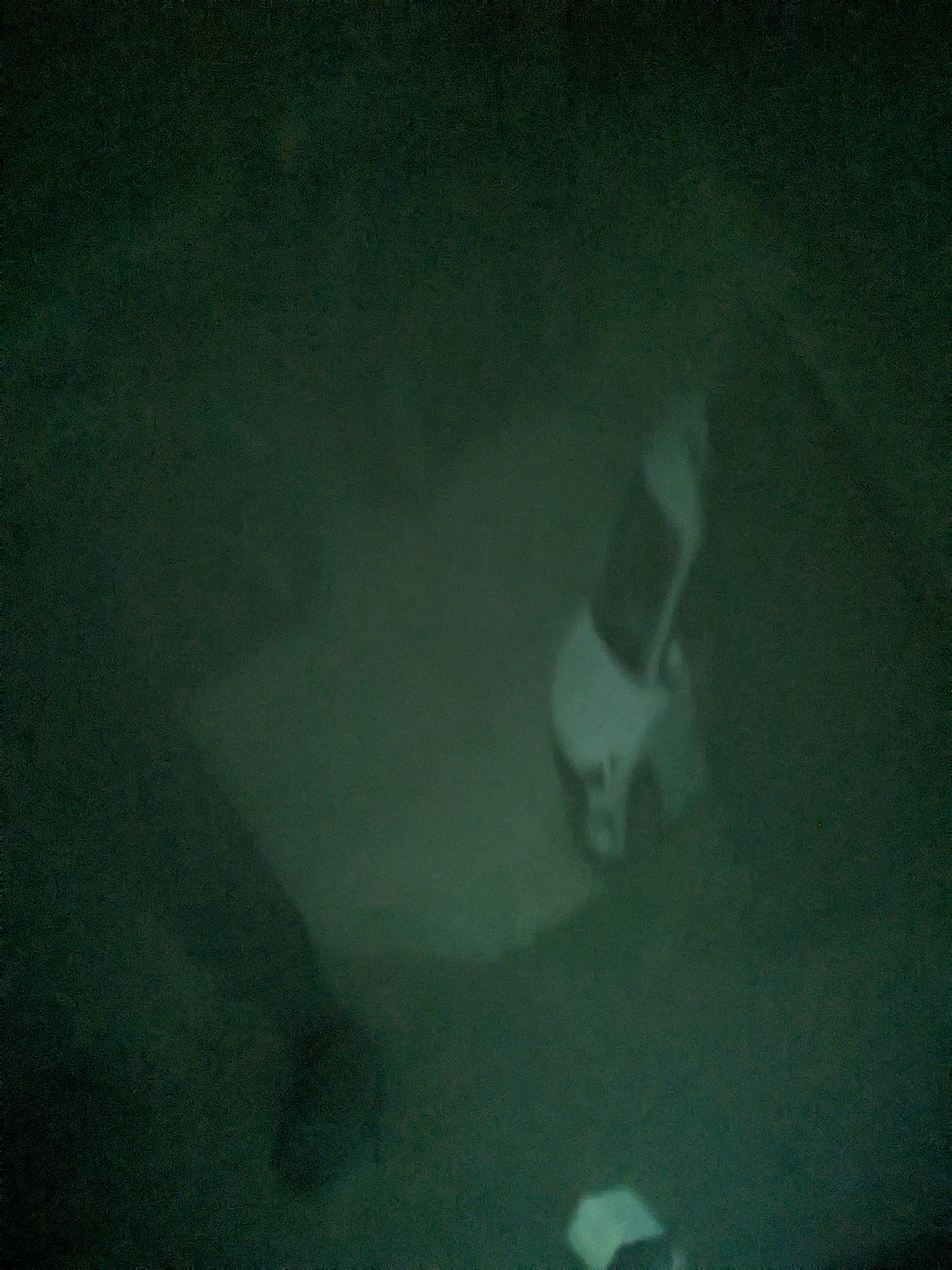This nighttime image features an overhead perspective of a dimly lit, possibly abandoned area or dark alley. The photograph is of low quality, adding to the overall darkness. At the bottom of the image, there is a distinctive white square object that seems to be a camera protruding from a building. The middle of the image reveals a lighter gray area, which appears to be a distorted road or parking pad. On the right side, a white vehicle, likely a van with a large windshield, is partially obscured by a dark black mass to its right. Only the front section of the vehicle is visible, from the driver's side rear-view mirror towards the front bumper and hood, with a barely visible black front tire blending into the gray background. The bottom of the image also shows a white rooftop object near the center. In the background, the top left section appears to have a wall or rocky structure, while the top right remains entirely black and blurry.